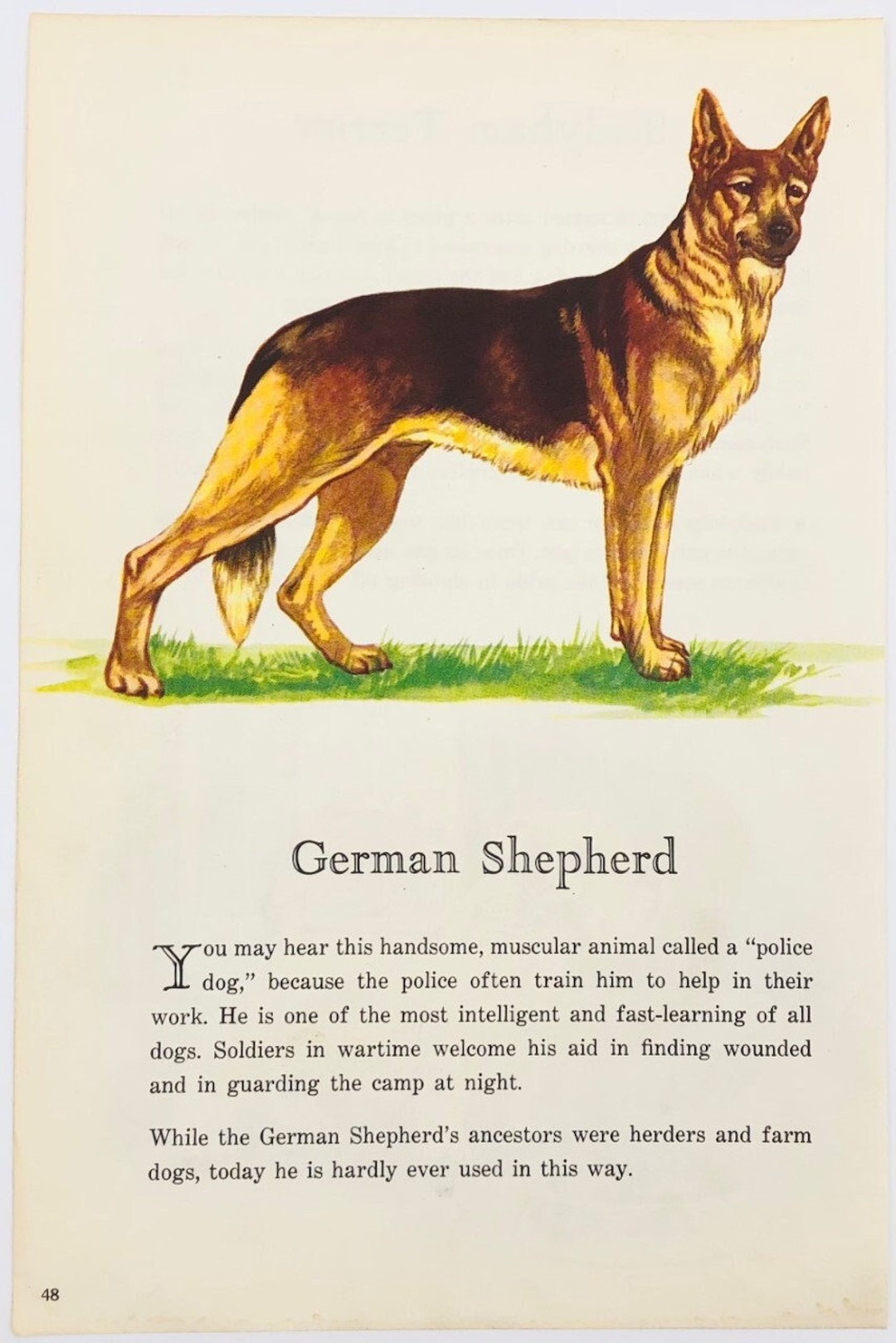The image appears to be a detailed illustration from a book or an educational poster, possibly from a museum exhibit or a zoo. It features a page numbered 48 with a beige or white background. At the top of the page is a finely drawn illustration of a German Shepherd. This large dog, known for its tan and dark brown coloring—its dark brown back contrasting with its golden underbelly—is depicted standing on grass and facing towards you, showing its right side.

Beneath the illustration, the caption identifies the breed as a German Shepherd. The accompanying text provides rich information about the breed, noting that it is often called a police dog due to its common use in law enforcement work. It describes the German Shepherd as one of the most intelligent and fast-learning dogs, valued by soldiers during wartime for its ability to find the wounded and guard camps at night. The text also mentions that although the German Shepherd's ancestors were herders and farm dogs, the breed is rarely used in this capacity in modern times.